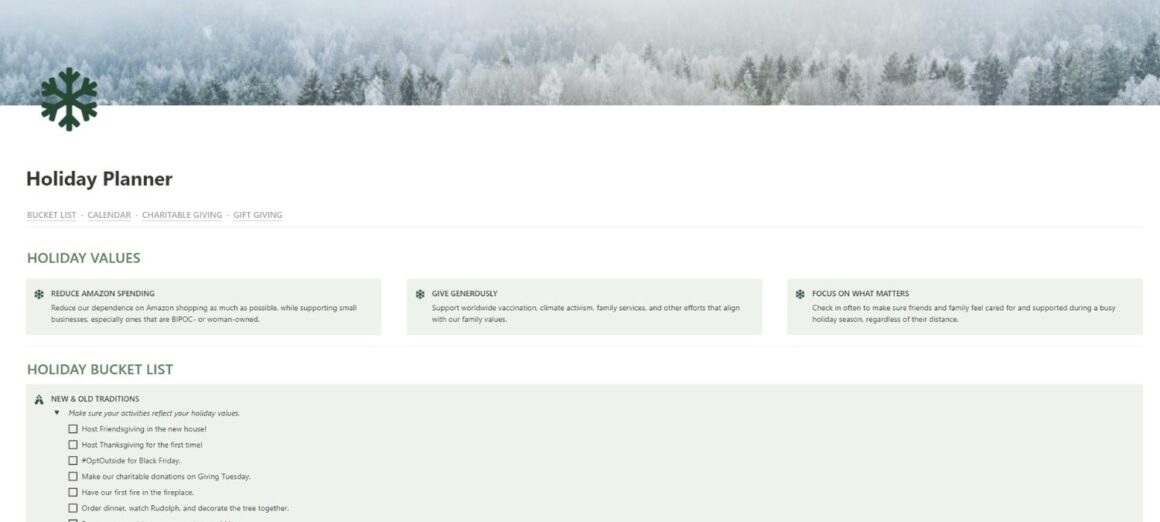This image depicts a serene winter landscape featuring a dense forest of pine trees, heavily blanketed in fresh snow, creating a picturesque, winter wonderland. On the left side of the image, there is a large green snowflake icon, beneath which the text "Holiday Planner" is prominently displayed. Further below, the text "Bucket List, Calendar, Charitable, Gift Giving, Holiday Values" outlines various themes and priorities for the holiday season.

The content is encapsulated within a gray box set against a white background and highlights a commitment to reducing reliance on Amazon by supporting small businesses, especially those owned by BIPOC and women. The text encourages generous giving and supporting worldwide climate activism, family services, and other causes aligned with family values. It also emphasizes the importance of maintaining connections with friends and family, regardless of their distance, during the busy holiday season.

The bucket list section encourages blending new and old holiday traditions and ensuring activities reflect personal holiday values. Some activities listed include hosting Friendsgiving at a new home, celebrating Thanksgiving for the first time, opting for outdoor activities on Black Friday, making charitable donations on Giving Tuesday, enjoying the first fire in a fireplace, ordering dinner, and watching "Rudolph" while decorating the tree together. This comprehensive plan aims to foster a meaningful and value-driven holiday season.